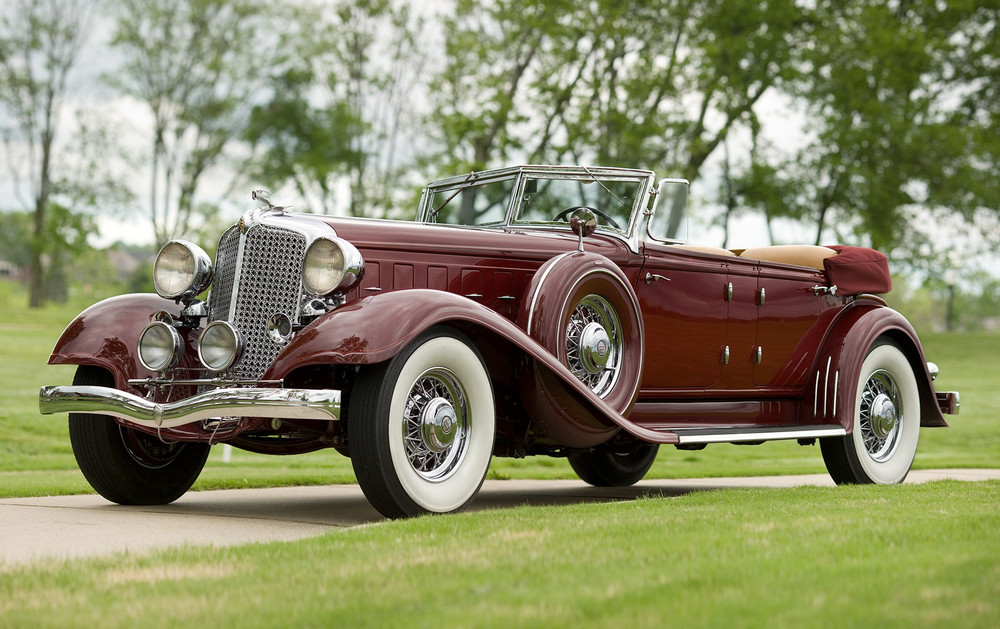This image vividly captures a striking burgundy classic convertible, reminiscent of a 1920s-era Rolls Royce. The vintage vehicle features prominent design elements, including four round headlights set above and below its sizable, intricately detailed chrome grille, which is adorned with fine square patterns. The long hood of the car contributes to its elegant and timeless appearance. The car's black tires are detailed with white trim and metallic spokes and notably include a spare tire positioned on the front fender, highlighting the era's automotive style.

This side profile shot also reveals beige trim accents on the convertible, suggesting that the roof is folded down, neatly stowed out of sight. The car sits poised in a serene nature setting, parked on a quaint path that resembles a golf course trail, surrounded by lush green grass and tall trees, suggesting a peaceful daytime outdoor scene. Despite the lack of drivers or additional context, this luxurious vehicle’s meticulously maintained condition hints at it being showcased, possibly at a car show or a judging event, evoking a sense of nostalgia for classic automotive craftsmanship.